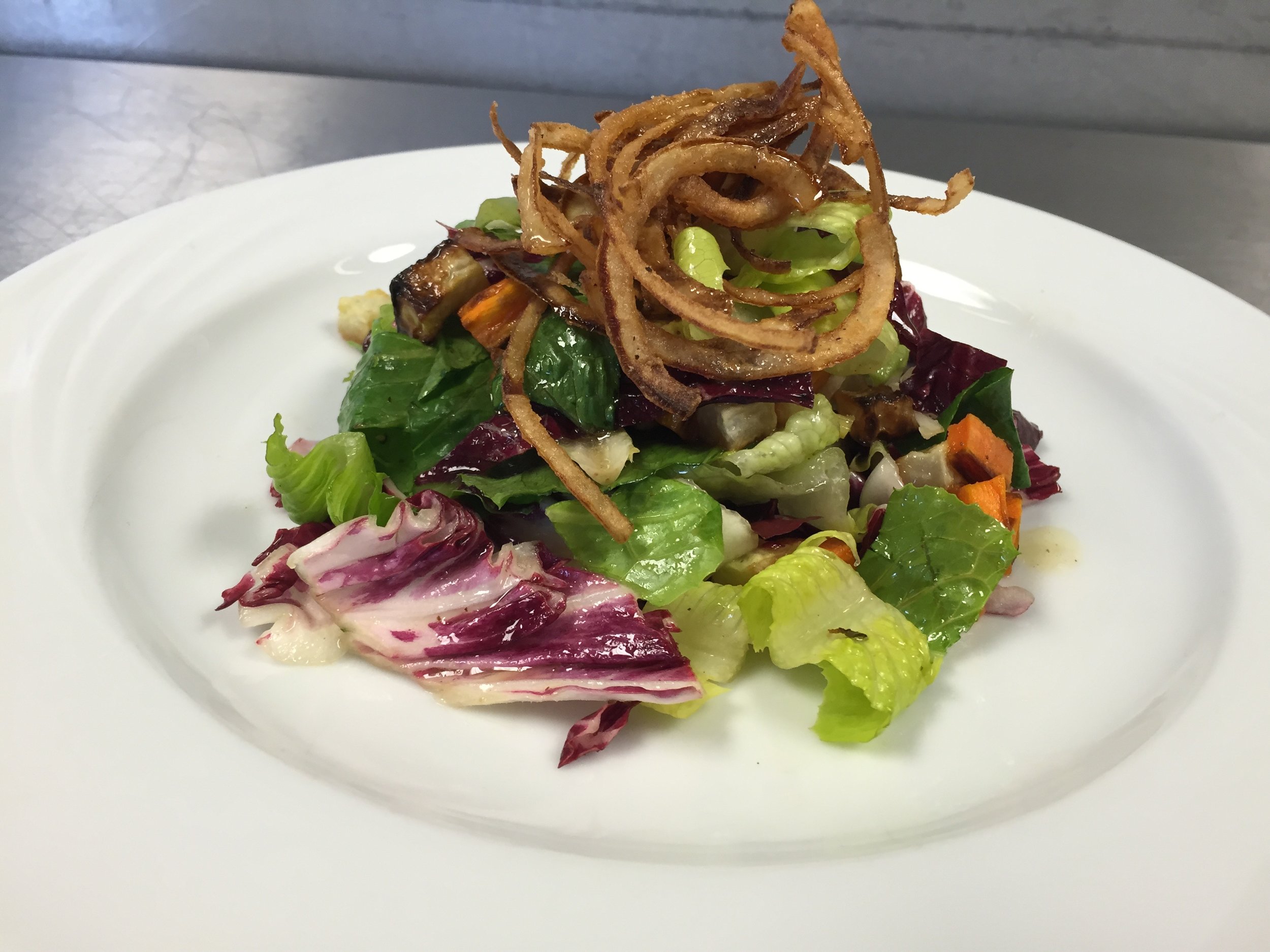This photograph features a close-up of a small mound of freshly prepared salad presented on a glossy, white, shallow, round plate that has a slight dip in the center. The salad itself comprises a mixed assortment of shiny, moist-looking light and dark green lettuce, some purple lettuce leaves, and bright orange carrot cubes, which could also be mistaken for sweet potatoes. Adding to the texture and flavor, there are fried golden-brown onion straws or potentially calamari on top, offering a distinct crispy garnish. Additionally, scattered among the greens, there are slices of red onions and potentially sautéed beets, all lightly coated in a seemingly clear dressing or oil, possibly vinaigrette or olive oil, giving the dish a healthy and appealing visual gloss. The plate is set on a black table against a backdrop of a gray, concrete-looking wall, with some hints of a kitchen environment, suggesting that the dish is yet to be served to a customer. The vibrant colors and the textural variety of the ingredients make the salad look both appetizing and aesthetically pleasing.